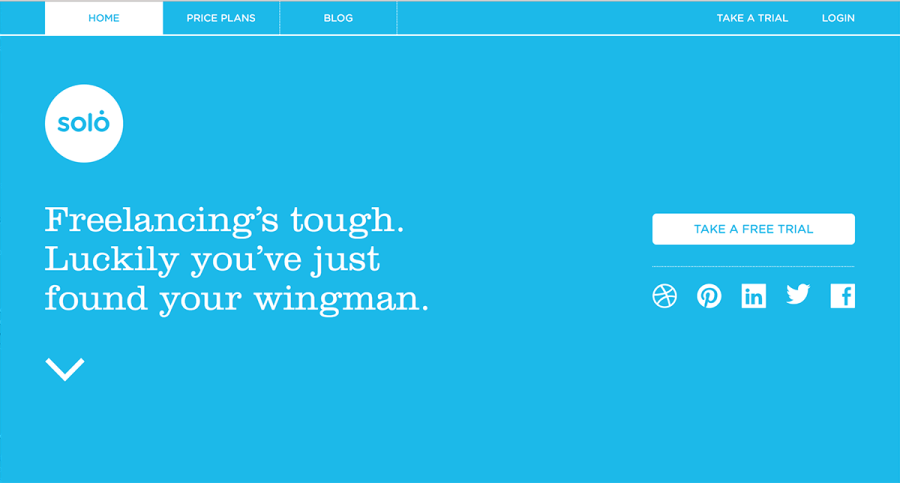The image features a partial view of a computer screen displaying a bright blue website. The website's navigation bar, situated at the top of the screen, includes several sections: "HOME," "PRICE PLANS," "BLOG," and, on the far right, "TAKE A TRIAL" and "LOG IN." All these options are written in white capital letters, except for "HOME," which is in blue capital letters highlighted by a white background, indicating it’s the currently active page.

In the upper left corner of the main section, there's a white circle enclosing the word "solo" in lowercase letters, featuring a unique accent resembling a dot above the letter "O," which appears to be the logo. Below the logo, a bold white text proclaims, "Freelancing's Tough. Luckily, you've just found your wingman." Directly beneath this, a white downward-pointing arrow suggests further content below.

Adjacent to the logo and text, there's a prominent white banner on the right. This banner displays the words "TAKE A FREE TRIAL" in blue capital letters. Under this area, icons for various social media platforms are aligned horizontally. These include Pinterest, LinkedIn, Twitter, Facebook, and an additional, unrecognized icon.

Overall, the layout is clean and straightforward, with a consistent blue and white color scheme that draws attention to key features and navigation elements.